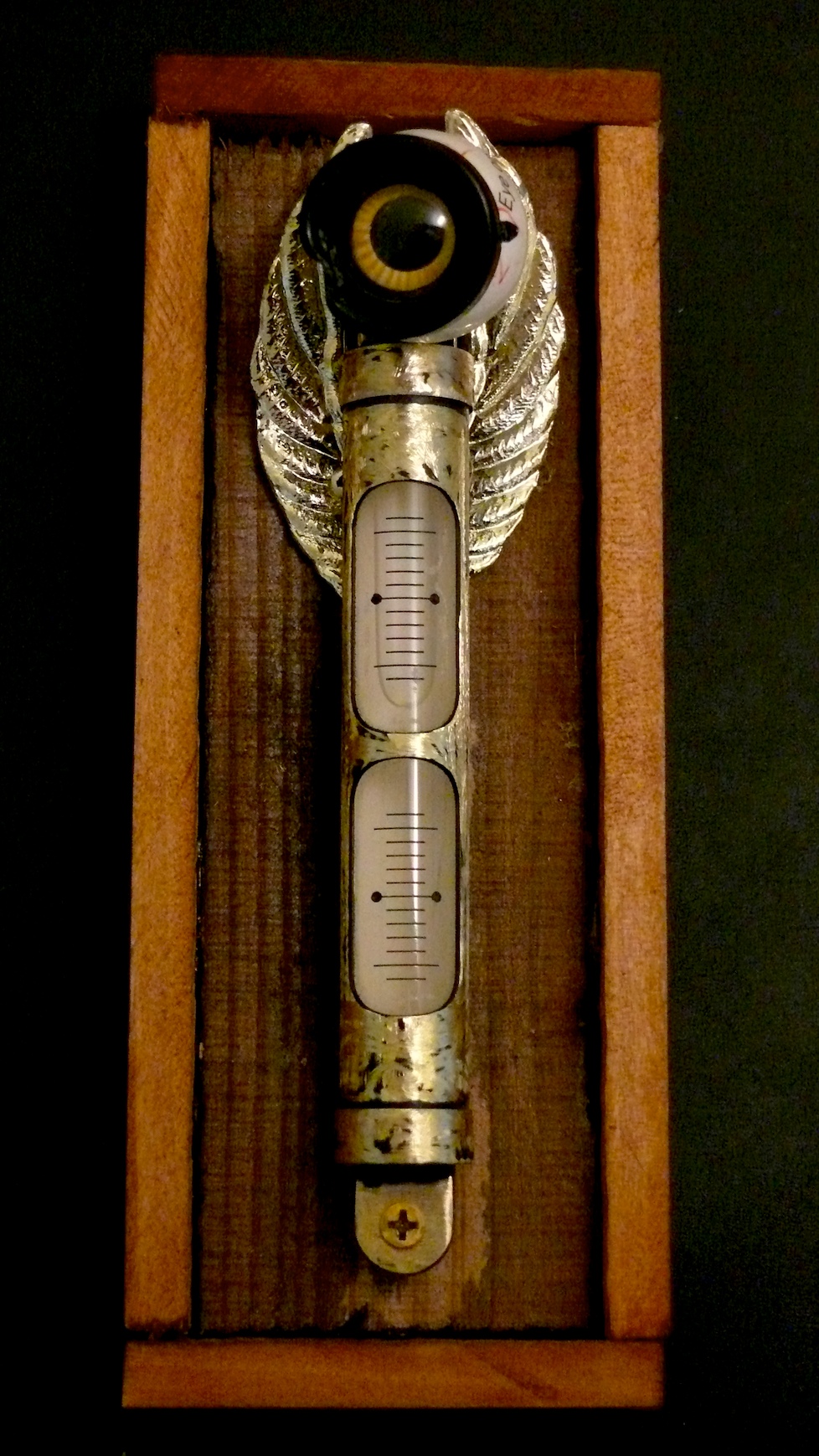The image showcases a vintage, wall-mounted thermometer affixed to a rectangular wooden backing. The wooden plaque has raised edges made from separate pieces of wood, exhibiting signs of wear and damage, particularly at the bottom. The thermometer itself lacks numerical markings; instead, it features black lines divided into two sections by a metal casing. Each section is distinguished by a thicker midline with circles at either end.

Mounted atop the metal casing is a decorative element: an artificial eyeball with wings. The eyeball has a yellow-orange iris, a black pupil, and a black cornea, giving it a striking appearance. The wings, long and slender, extend vertically from just above the midline circles to slightly above the eyeball. The metal casing shows some rust, adding to the vintage charm of the piece.